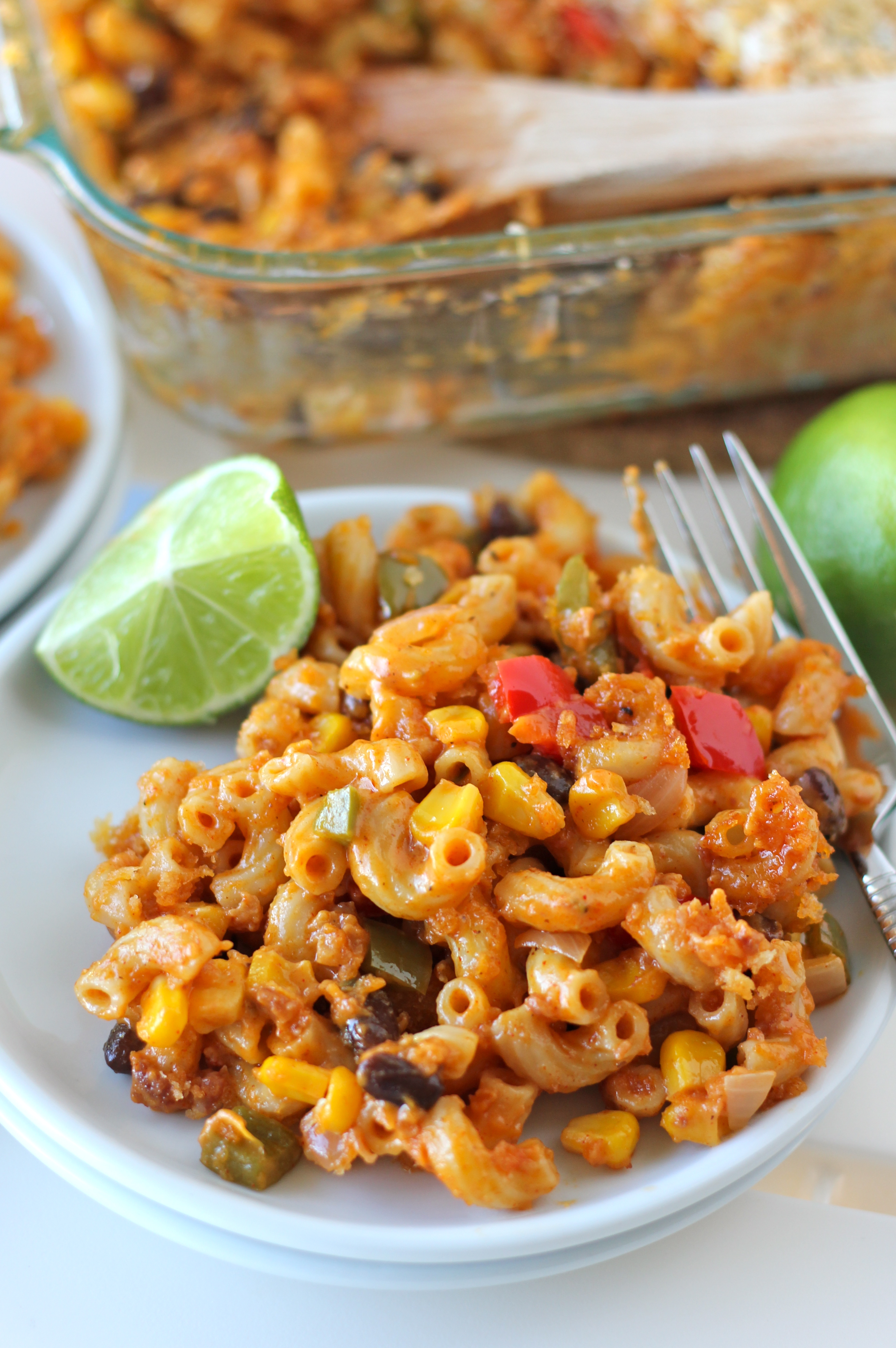A bright and detailed photograph showcases a shallow, white-rimmed bowl containing a dish of curved macaroni pasta, reminiscent of mac and cheese with a reddish-brown sauce. The pasta is adorned with corn, chopped tomatoes, and possibly green peppers and black beans. A lime wedge rests on the left edge of the plate, yet to be squeezed, while a whole, uncut lime is visible to the right. Partially visible on the right side, the silver tines of a fork indicate that the meal is untouched. The background reveals a clear glass Pyrex casserole dish with a large whitish scoop-type utensil, possibly wooden, sticking out. A small section of another bowl is slightly out of focus to the left of the casserole. The setting includes a white tablecloth, enhancing the visual appeal of the dish.